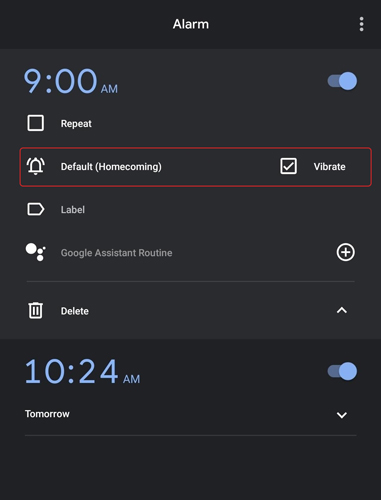This is a detailed screenshot of an alarm setting interface on a mobile device, which has a black background. At the top, an alarm icon is visible, indicating the alarm page. A 9:00 AM alarm time is prominently displayed in blue. Next to it, there is a blue toggle button to activate or deactivate the alarm. Below the time display, a "Repeat" option is shown, but the box is not checked, indicating the alarm is set for a one-time event.

Further down, there is a "Notification" section that shows a default bell icon for notifications. Here, a box is checked for the "Vibrate" option, indicating the device will vibrate when the alarm goes off. An option labeled "Label" allows for customizing the alarm name, while the "Google Assistant Routine" setting is also available with a plus sign next to it, indicating you can add a new routine.

At the bottom, there's an option to delete the alarm. Another alarm is listed below for 10:42 AM, which is enabled and scheduled for the next day.